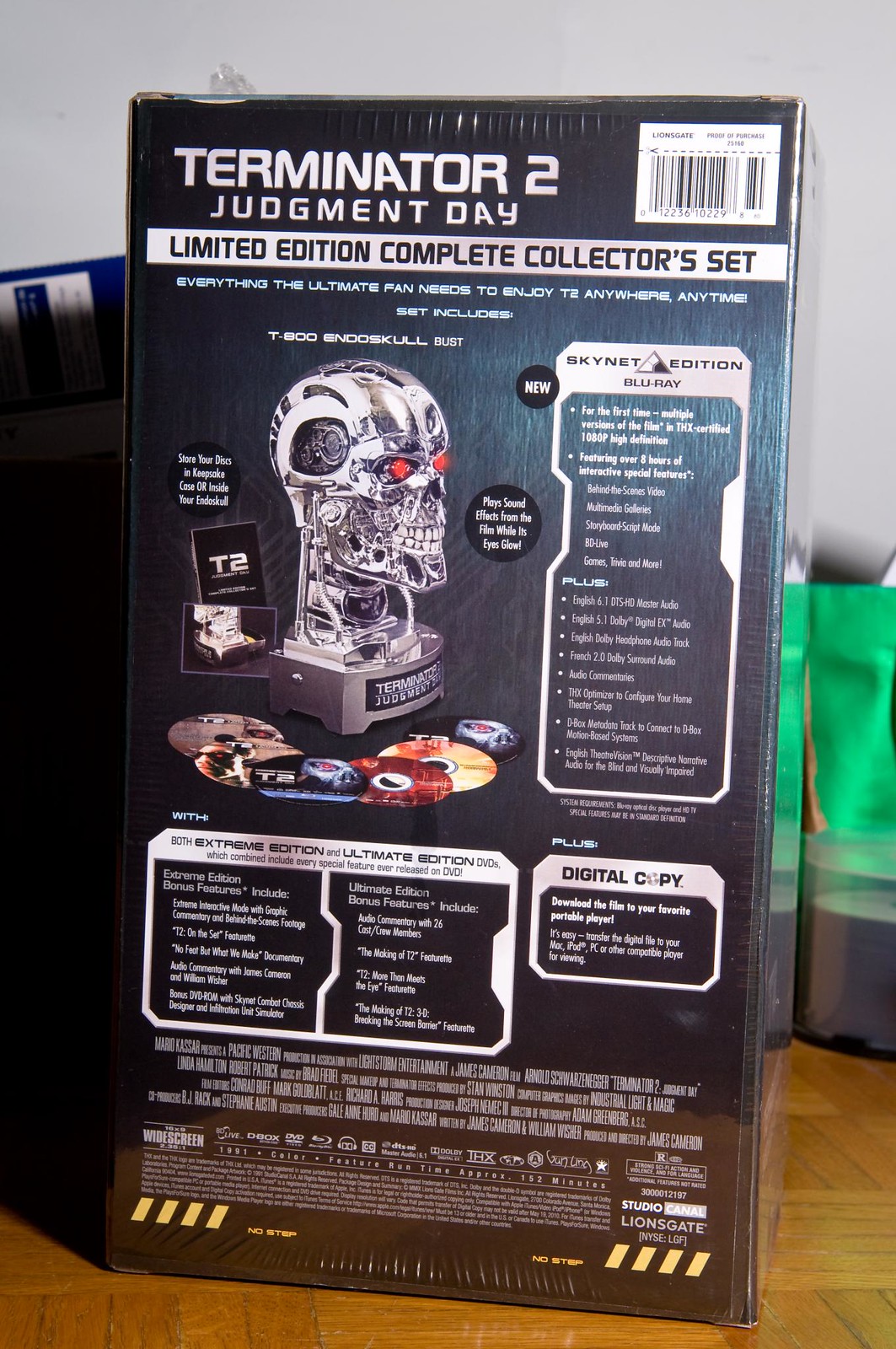The image depicts a detailed and visually striking Terminator 2: Judgment Day Limited Edition Complete Collector's Set. Prominently featured on the back of the box is a striking image of the iconic T-800 Endo Skull Bust with its metallic texture and eerie red eyes. The box emphasizes it includes six DVDs, showcasing various editions of the film: the Skynet Edition Blu-ray, Extreme Edition, and Ultimate Edition, among others. This collector's set is packed with over three hours of interactive special features in TMX certified 1080p resolution. Additionally, there's a digital copy option, allowing fans to download the film to portable devices like Knox iPads and PCs for easy transfer. The packaging itself is primarily black and green, adorned with a plethora of text such as "Terminator 2: Judgment Day," "Limited Edition Complete Collector's Set," and "Everything the Ultimate Fan Needs to Enjoy, T2, Anywhere, Anytime." The box includes a barcode in the top right and mentions Lionsgate Studios, hinting at the production company involved. The setting appears to be either a room or a house, adding to the personal collector's vibe.